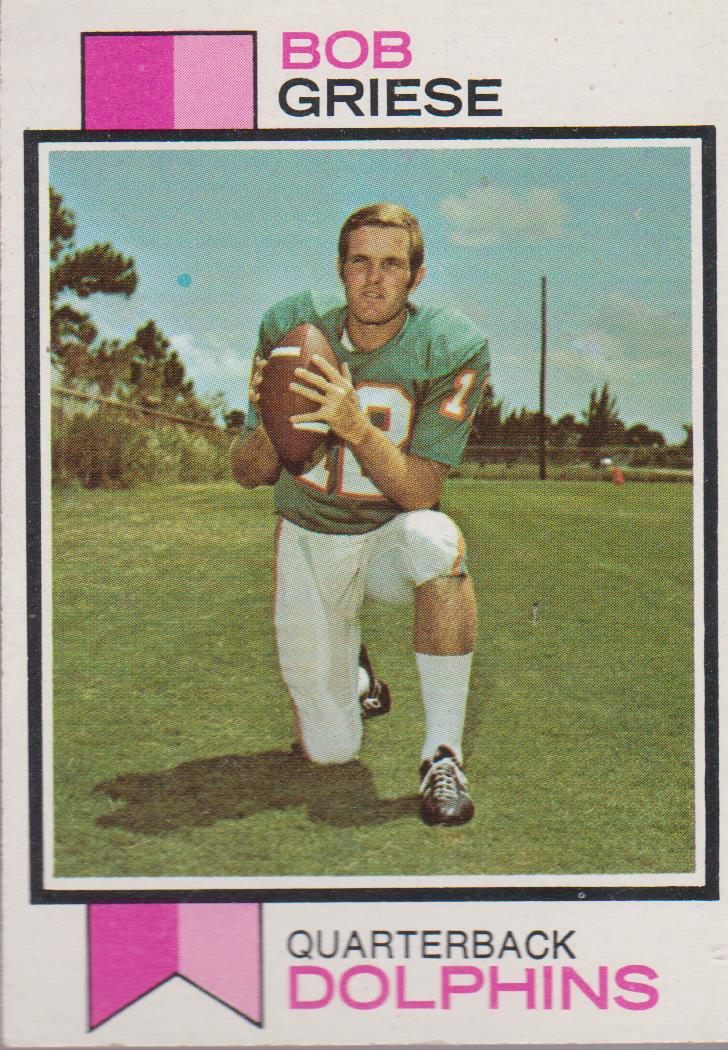This image is a detailed scan of a vintage football trading card featuring Bob Griese. The card prominently displays his name at the top, with 'Bob' in pink and 'Griese' in black lettering. A striking pink and purple two-tone ribbon extends behind the photograph and ends with a pointed tip at the bottom. The center of the card showcases Griese kneeling on a grassy field under a clear sky with white clouds. He is dressed in a green number 12 jersey with an orange border, white socks, and black cleats. His left knee is up with his foot firmly on the ground, elbow resting on the knee, and his right knee bent, touching the ground. Griese holds a football with both hands as if poised to hike it. The bottom of the card features the text 'Quarterback' in black and 'Dolphins' in bold pink letters, all set against a white background with a thin black border enclosing the entire image. The scene behind Griese suggests an outdoor setting with trees rather than a professional stadium.